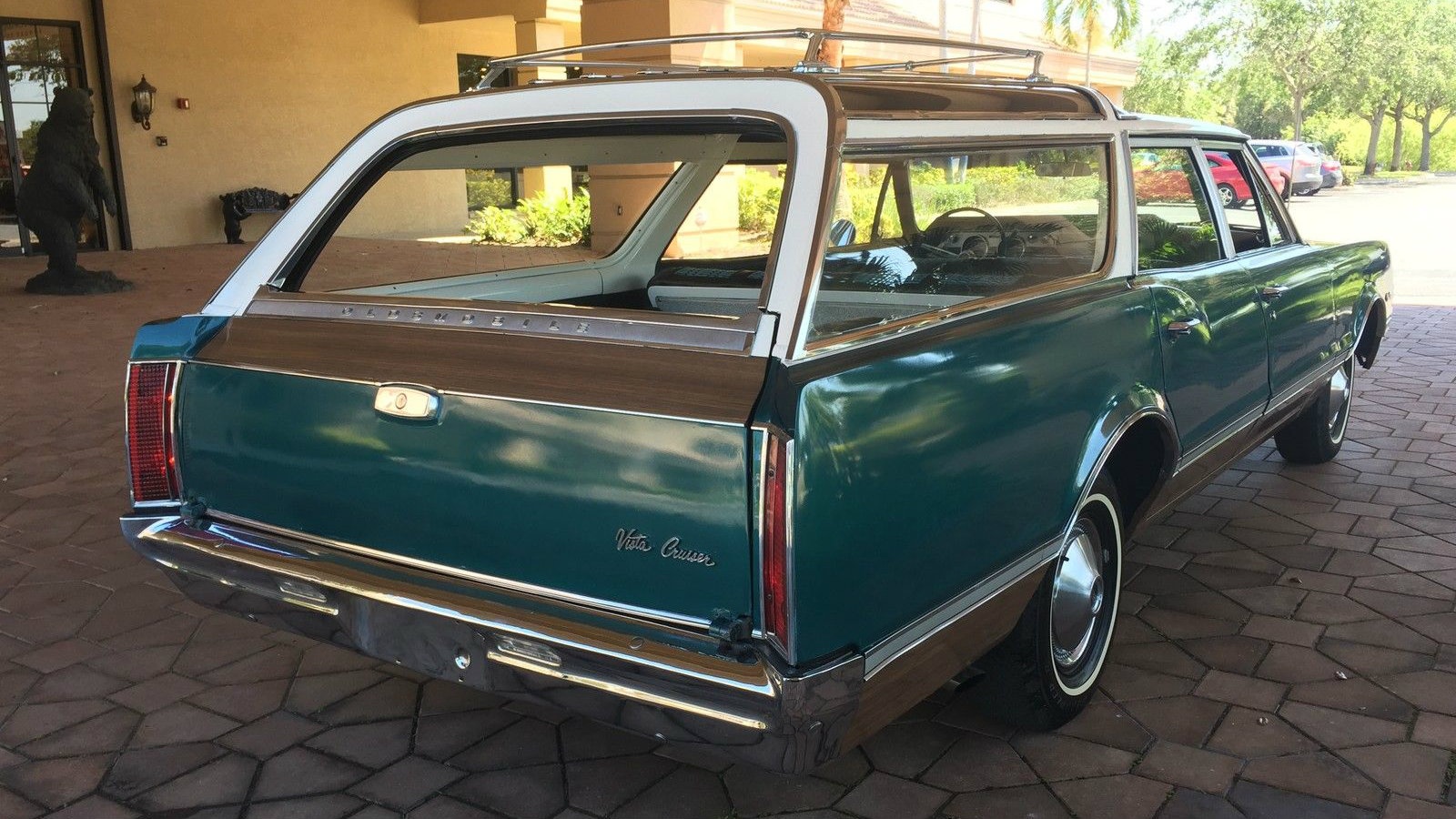The image captures a vintage 1960s or 1970s Vista Cruiser station wagon in an idyllic tropical setting. The car, characterized by its distinctive aqua greenish-blue color with wood paneling trim, boasts a shiny, glossy finish that reflects the sunny surroundings. Its roof is white and features a luggage rack. The vehicle is parked on a patterned or cobblestone driveway under an awning, likely at the entrance of a hotel or resort, suggested by the presence of a peach stucco building, a black wrought iron bear statue, and a bench in the background. This old-timey station wagon has chrome trim accents, whitewall tires with silver hubs, and a noticeable lack of a license plate and rear windshield. The trunk area appears covered, adhering to the traditional design of the era. The overall perspective shows the car from the back and slightly diagonal to the driver's side, with the right side and taillights clearly visible. Additional cars are parked further in the distance, enhancing the vintage vacation ambiance.